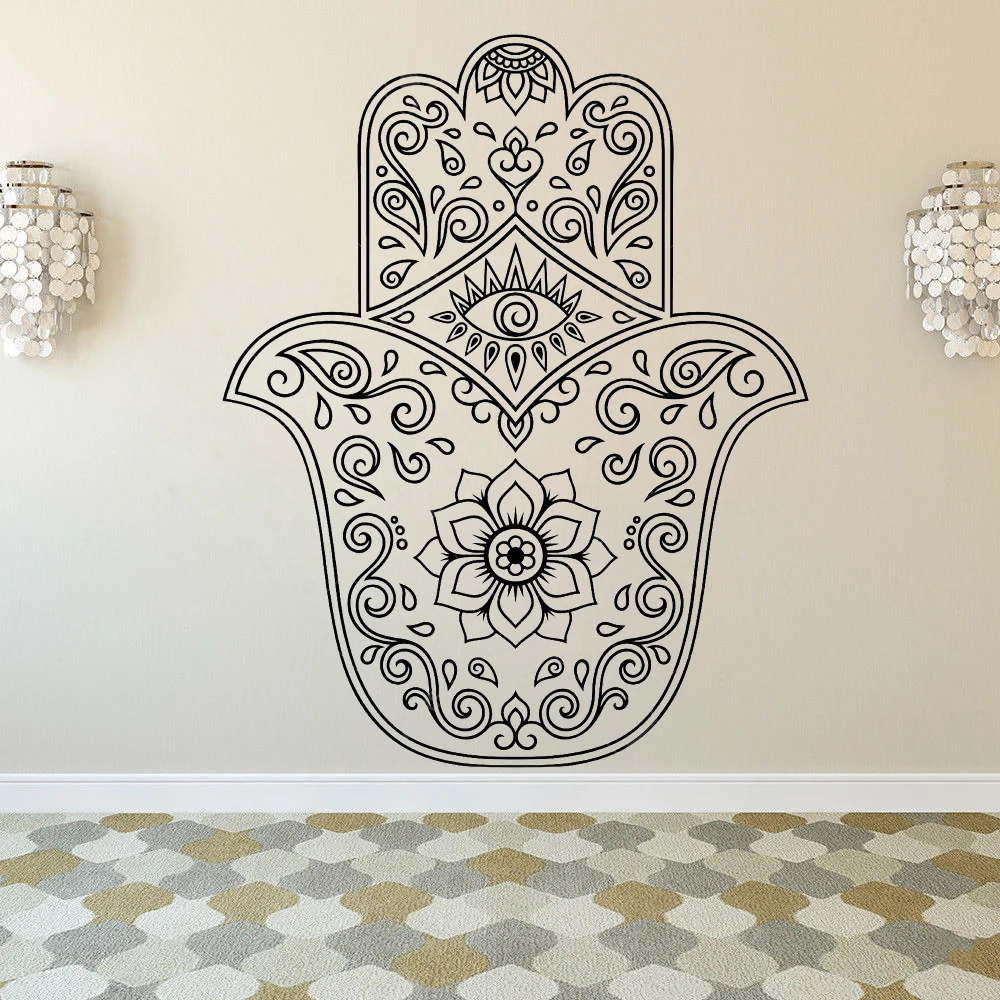The photograph depicts a section of a home with a cream-colored wall adorned by a highly detailed, black ink mural. The mural, outlined in black, resembles a hand with a central eye, complete with eyelashes, in the palm. Below the eye is a filigree pattern incorporating a lotus flower, and above, intricate elements evoke a mandala design. On either side of the mural, wall sconces with hanging circular adornments add a touch of elegance. The floor features a wall-to-wall carpet with a striking geometric pattern of alternating bright shapes in white, gray, olive green, and brown, resembling a mosaic. The overall scene blends elements of artistic expression with homey comfort.